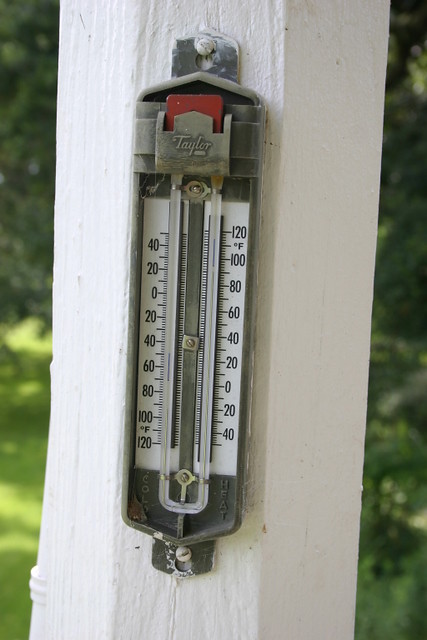The image captures an outdoor scene with lush, leafy greenery on both the left and right sides, creating a natural, verdant backdrop. In the center of the composition stands a white wooden structure. Prominently featured on this wooden surface is a vertical thermometer. The thermometer is secured with thumbtacks at both its top and bottom ends.

The thermometer itself has several noteworthy details. At the top, there's a label that reads "Taylor," likely denoting the brand. Below this label, there's a red square marking the current temperature. The temperature scale on the left of the thermometer ranges from 40 to 120 degrees Fahrenheit, while the right side mirrors this scale with 120 at the top and 40 at the bottom. Small dashes mark increments along both scales. A metallic strip runs vertically through the center of the thermometer, connecting it to the wooden backing. The overall context of the image suggests a serene, outdoor environment, where the weather and temperature play a noticeable role.